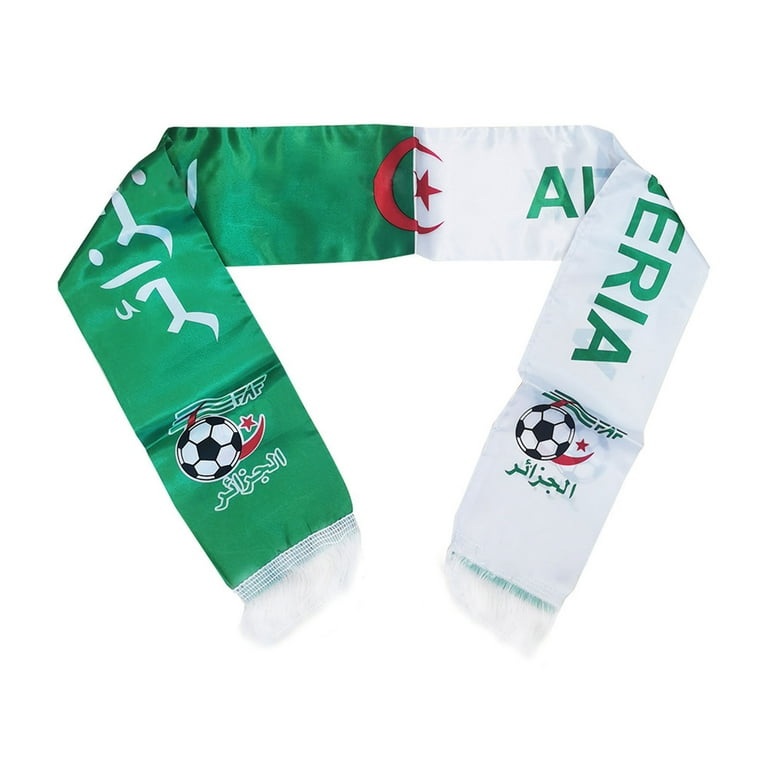The image features a scarf commonly worn by football fans, showcasing a design that hints at support for the Algerian soccer team. The scarf is divided horizontally, with the left side being a shiny, light green and the right side being a sheer, shiny white. Both ends of the scarf are adorned with frayed tassels. 

On the green side, there's white text and a prominent image of a soccer ball, accompanied by what appears to be Arabic writing. There's a notable red crescent moon and a five-pointed star, symbolizing elements of the Algerian flag, featured on both sides and interspersed with the soccer imagery.

The white side mirrors this design with green text and similarly includes a soccer ball and Arabic writing. The scarf also features the letters "F-A-F," possibly standing for Fédération Algérienne de Football. Despite some folding obscuring parts of the text, it seems likely that the scarf references Algeria, given the repeated visual cues and textual hints. The overall design is vibrant and celebratory, embodying the spirit and pride of Algerian football fans.